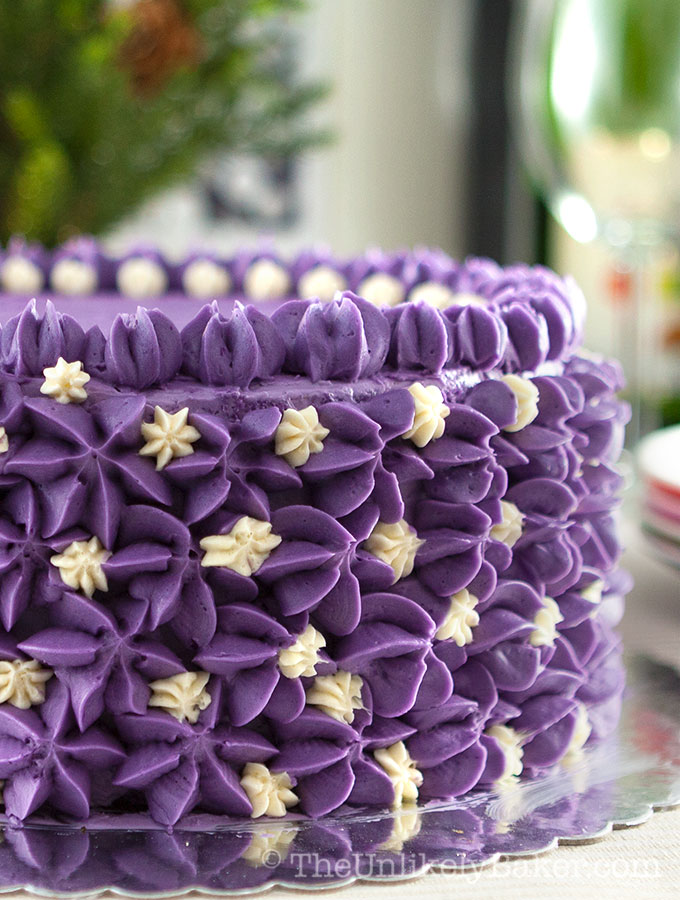A beautifully decorated cake sits in the center of the image, resting on a thin, reflective silver cake platter with scalloped edges. The cake is entirely covered in a rich purple icing, intricately fashioned into various flower designs. Larger, connected purple flowers form a ring around the entire cake, while smaller white frosting flowers are interspersed amidst them, creating a delicate contrast. The top of the cake is adorned with more piping, featuring lighter purple flowers around the edges and additional small white flowers. The backdrop is slightly out of focus, revealing a domestic setting with a window on the right and a small plant with a seemingly dying flower on the left. There is also an empty wine glass in the top right corner, a small plant in the top left, and the edge of a patterned cup on a white saucer with red, pink, and green stripes just to the right of the cake.